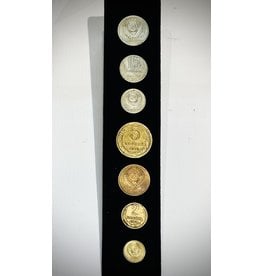The image showcases a set of coins arranged on a white background with a grayish tint overlay. The collection includes seven coins placed within a black strip. At the top, there are three silver coins, followed by a larger gold coin in the center, which prominently features the denomination "5". Beneath this central coin, there are three more coins: two with a gold hue and one with a coppery-tone. The coins' arrangement and varied colors create a visually striking display, despite the overall low resolution of the image.